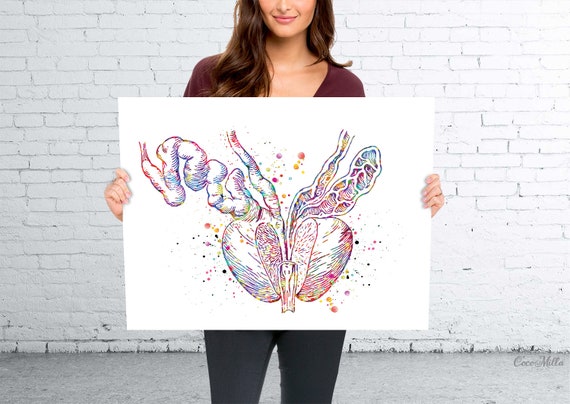This is a detailed photograph of a woman standing against a painted white brick wall, on a gray cement floor. The woman's face is visible from the nose down, and she has long, curly, wavy brown hair that extends beyond shoulder length. She is dressed in a burgundy v-neck t-shirt and gray jeans. She is holding up a white poster board, which prominently features a large, colorful, abstract illustration that resembles internal organs. The drawing depicts a split-open apple-like shape with various tubes extending from it, somewhat resembling intestines. The vivid illustration is splattered with a diverse palette, including shades of yellow, blue, red, orange, purple, and a touch of black. In the center of the drawing, there is an element that looks like two kidney beans connected by a ureter, with colorful dots surrounding the lower part of the piece. The setting of the photograph is ambiguous regarding whether it's indoors or outdoors, as there is some natural light, but it is not definitive.